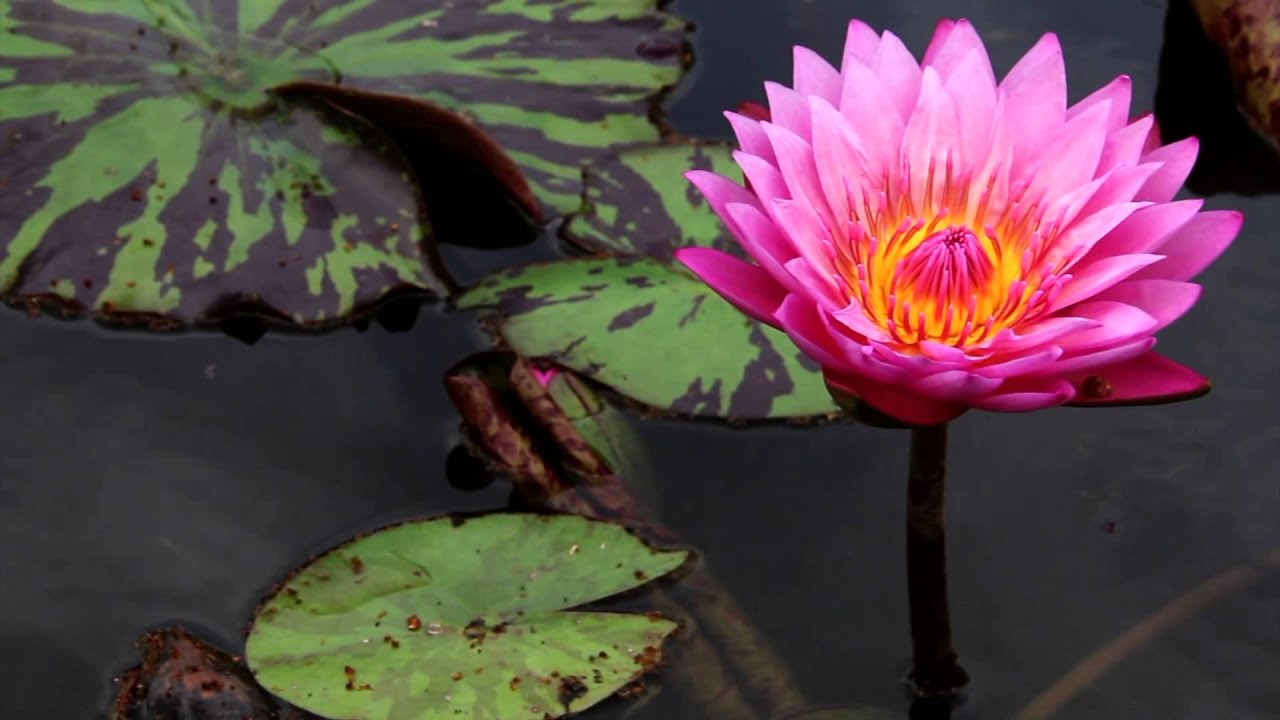The photograph is a horizontally oriented, rectangular snapshot taken outdoors during the daytime, looking down into a pond-like body of water. Dominating the right side of the image is a large, fully bloomed pink lotus flower. The lotus has a vivid center with shades of orange and yellow, surrounded by a dome of pink and yellow stamens, and about 30 to 40 thin pink petals that come to long points. Below the lotus, dark gray water is visible, speckled with sticks and twigs.

To the left of the lotus, there are three distinct lily pads, varying in size and color. The smallest lily pad is near the bottom left, predominantly green with a few brown splotches. Above and to the right of this pad is a slightly larger one with additional brown striations. The largest lily pad is situated further up and to the left, exhibiting more pronounced brown splotches and some tearing. The water beneath the lily pads appears dark and murky, contrasting with the vibrant flora above.